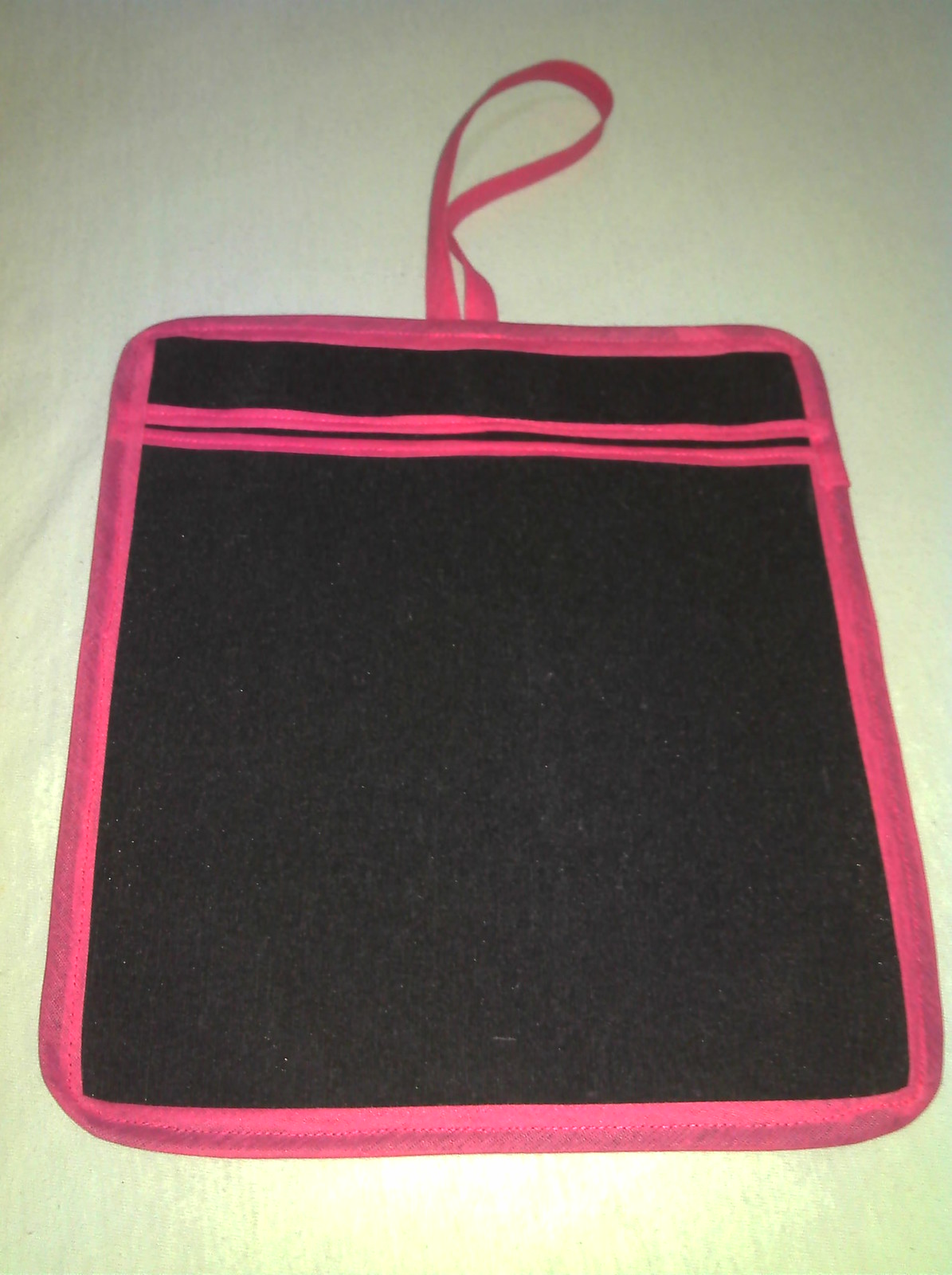The image depicts a rectangular, flat, zippered storage bag, likely designed for holding school supplies or small papers. The bag is primarily made of black fabric, with bright hot pink trim outlining its edges and forming two horizontal lines close together across its front. A pink fabric handle is attached at the top, extending upwards before doubling back to connect with the bag. The bag appears quite thin and possibly intended for items like pencils or a few sheets of paper. It rests on a slightly yellowed white fabric background, resembling a tablecloth, suggesting the bag is on display.